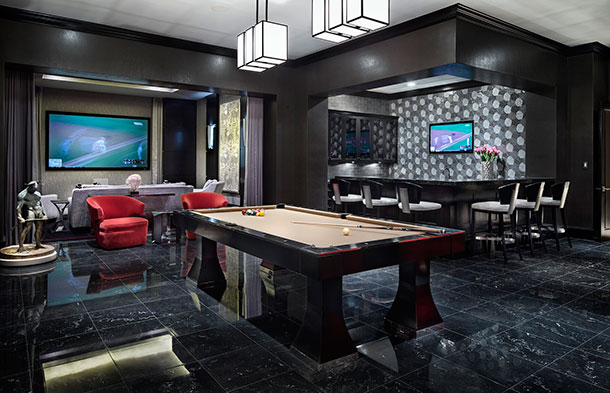The image showcases a meticulously designed space that could be inside a bar, hotel lobby, or a man's exclusive lounge. The room features glossy black tile flooring adorned with white and gray streaks that add a modern touch to the elegant ambiance.

In the back corner, there's an open curtain revealing another room. This room houses a state-of-the-art flat-screen TV mounted on the wall, currently displaying a live baseball game. Positioned in front of the TV is a comfortable couch, which is complemented by two plush red velvet chairs situated behind it, creating a cozy viewing area.

Towards the front of the room stands an artistic statue depicting a man holding a stick, contributing to the room's sophisticated decor. Adjacent to the statue on the right is a stylish metal pool table with a tan playing surface. The balls are neatly racked, and a pool cue rests on top, ready for a game.

On the back right side of the room is a well-appointed bar area, arranged in a V shape with six inviting chairs lined up around it. Behind the bar, a cabinet is filled with an assortment of liquor bottles, enhancing the room's luxurious feel. Above the bar, a smaller TV, also tuned to the same baseball game, ensures guests won't miss any action while enjoying their drinks.